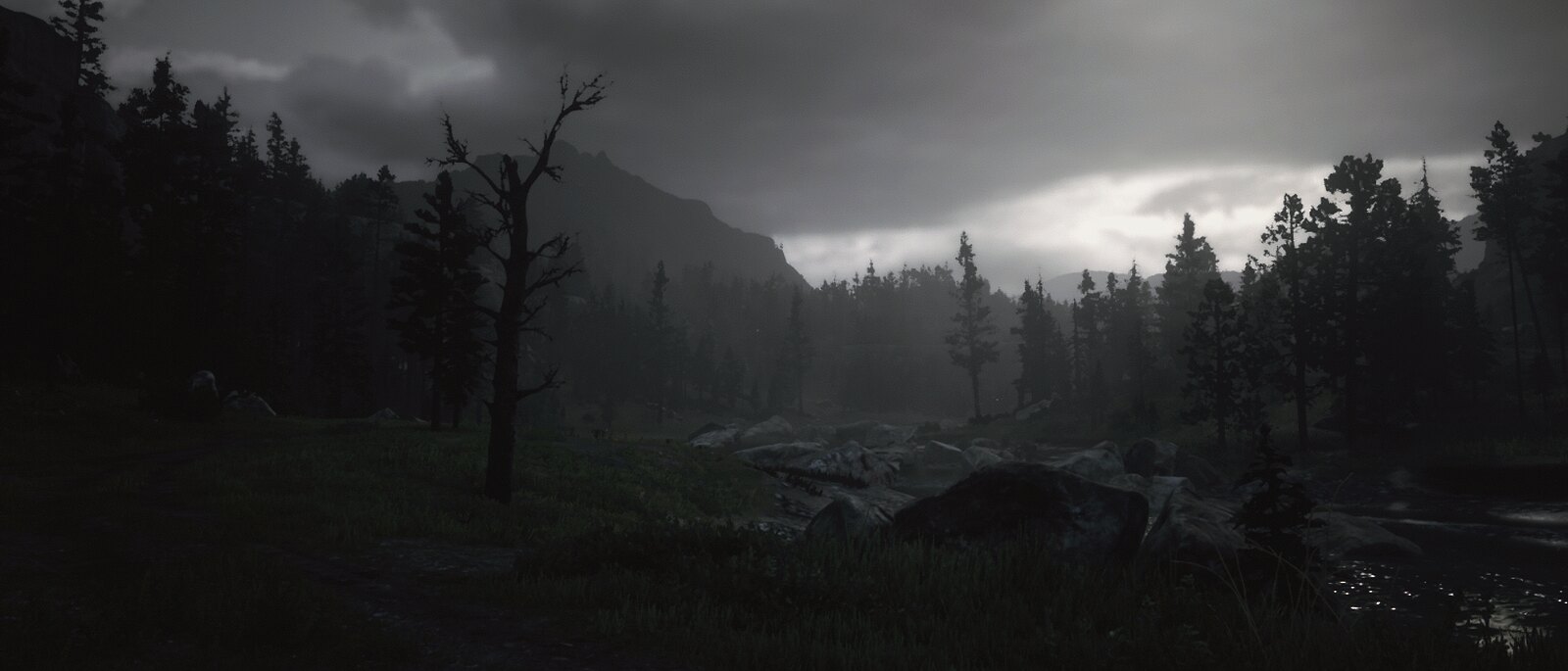A striking black-and-white, potentially computer-generated image captures a dramatic landscape beneath a tumultuous sky filled with dark clouds. A small swath of lighter, almost white sky suggests a glimpse of sunlight breaking through the overcast. The background features rugged, craggy mountains, adding a sense of depth and scale to the scene. In the mid-ground, a dense forest of tall pine trees extends towards a clearing. This open space reveals a flowing river, its bank strewn with a jumble of rocks and boulders. Sparse patches of grass, barely distinguishable in the grayscale palette, hint at hints of green, lending a touch of subtle life to the otherwise monochromatic vista.